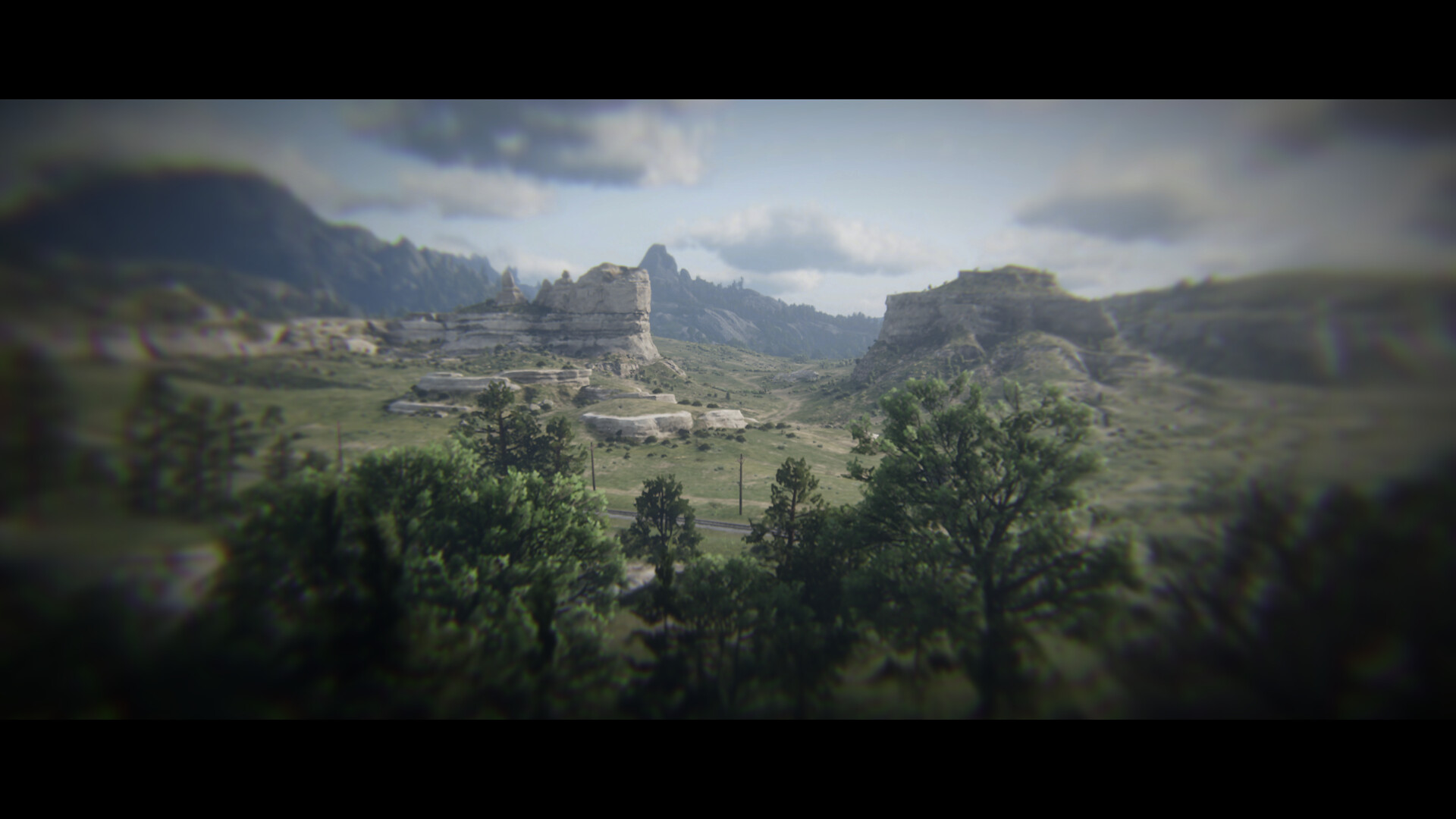The image captures a stunning outdoor scene that merges natural beauty with an almost surreal quality. The sky is a blend of pale blue and white, dotted with thick clouds, some of which are dark gray and infused with varying degrees of thickness. Below this dramatic sky lies a series of jagged mountain peaks, cascading down into a hilly, grassy landscape adorned with tall, jagged rock formations. These rocky outcrops are predominantly covered in grass, and sprinkled with lower-level trees. 

In the immediate foreground, the scene shows a mix of lofty trees, including oaks, maples, and evergreen pines. Between these trees and the rock formations, a black asphalt road snakes through the valley, faintly visible along with its accompanying telephone poles. The high-quality image appears almost digital, with black cinematic bars on the top and bottom adding to its polished feel. The outer edges of the image are slightly blurred, directing focus toward the center and enhancing the overall ethereal effect of this picturesque landscape.